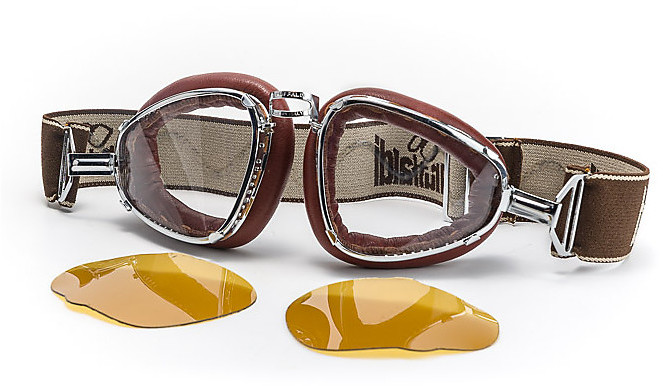The image features a pair of vintage-looking flight goggles with a classic design. The goggles have a sturdy metal construction and feature a dark maroon color with cushioned rims around the lenses, ensuring comfort and wind protection. The cushioning is distinctly red, adding to the retro aesthetic. The lenses are currently clear but come with additional yellow-tinted lenses that can either clip on or replace the clear ones for versatile usage. The goggles are held in place by a dark brown, stretchy strap that resembles those used for headlamps and is adjustable for a secure fit. The strap's inner side is tan and gray, featuring a logo, possibly reading "IBISTUIL." The entire setup, including the extra lenses, is laid out on a white background, highlighting the goggles' intricate details and robust construction.